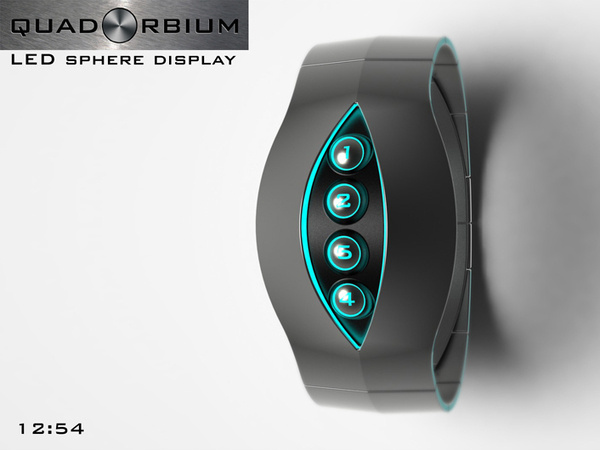This close-up image depicts a futuristic, high-tech smartwatch, showcasing an artistic and innovative design. The watch itself features a sleek, matte gray finish and highlights a unique, elongated, oblong, leaf-like centerpiece that glows with aqua blue LED lighting. Embedded within this shape are four buttons with undecipherable icons, outlined in a light aqua blue color, which could possibly function as control knobs. Prominently displayed in the upper left corner of the image is a logo reading "Quad RBM", with the text "LED Sphere Display" underneath it. The lower left corner indicates the time as 12:54. The background of the image is plain white, ensuring the focus remains on the cutting-edge design of the smartwatch.